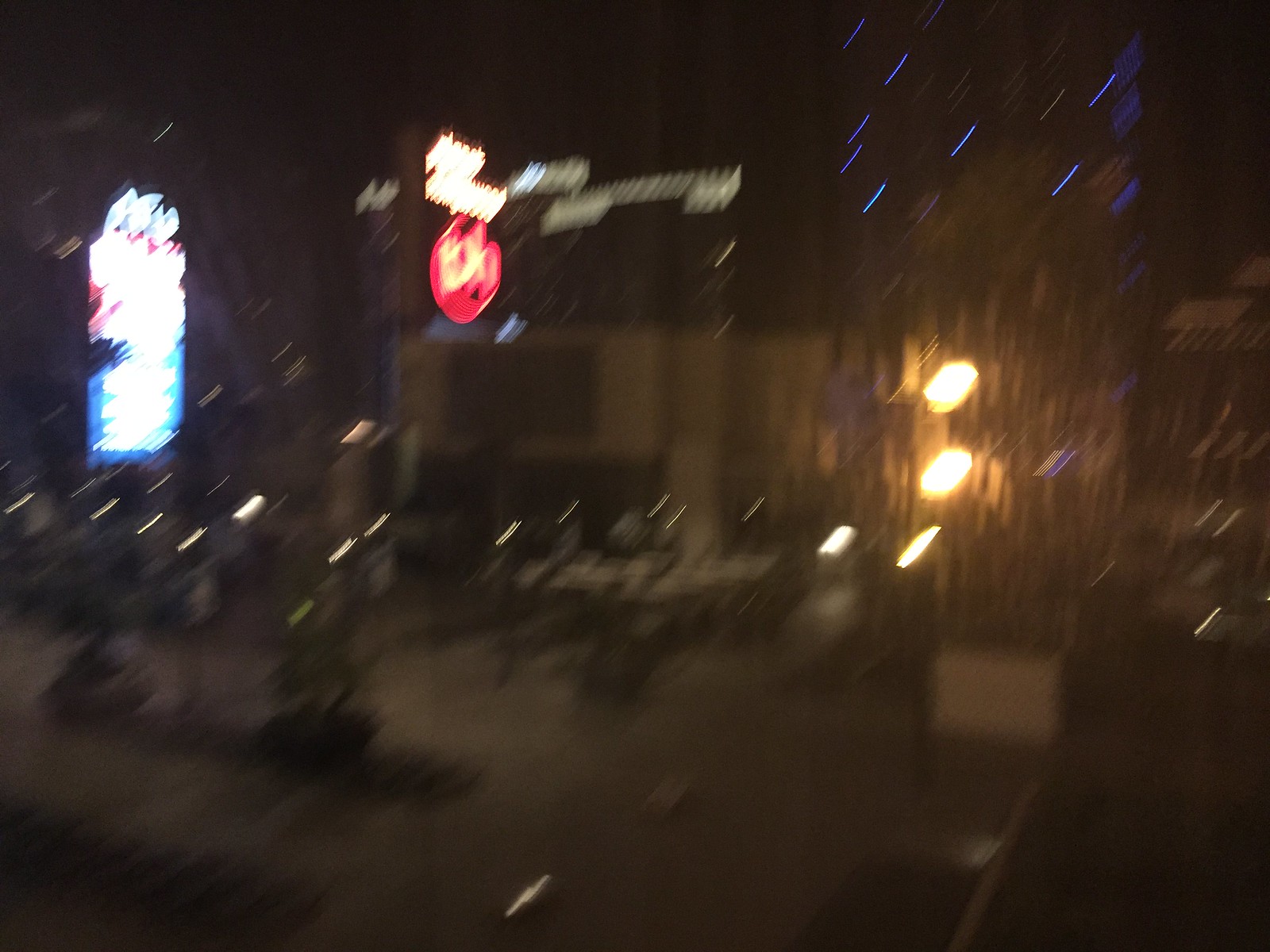This photograph appears to capture the interior of a building, albeit slightly blurry and out of focus, likely due to the photographer's movement upwards to the right during the shot. The scene is predominantly dark in the lower half, with some areas nearly obscured in shadow. 

On the right-hand side of the image, there is a seating area adjacent to what seems to be a stage. Two very bright lights are positioned on the right, casting an intense glow. The center left and far left of the image feature several neon signs, though the details of these signs are unclear due to the blur. 

One significant sign in the upper left is approximately rectangular, displaying a blue and white section below and a red and white section above. Another noteworthy element is a heart-shaped image in the center left, predominantly red with some yellow inside, and potentially some white text above it. Light streaks, predominantly in the upper portion of the photograph, add to the overall sense of motion and haziness.